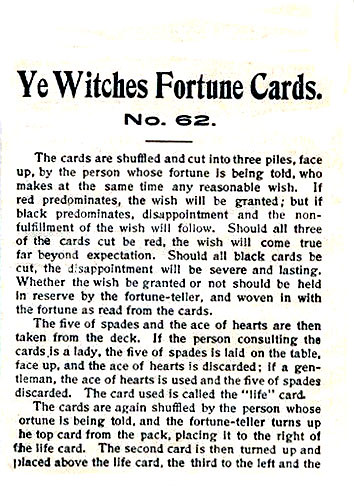The image depicts the exterior of a vintage playing card box labeled "Ye Witches Fortune Cards, No. 62." The front of the box features several paragraphs of instructions for performing a fortune-telling ritual. According to the instructions, the cards are shuffled and divided into three face-up piles by the seeker, who makes a reasonable wish in the process. The color predominance of the cards reveals the outcome of the wish: a red majority signals fulfillment, while a black majority indicates disappointment. If all three cards cut are red, the wish will be granted beyond expectations, but if all are black, the disappointment will be severe and lasting.

Further instructions detail the use of the Five of Spades and the Ace of Hearts based on the seeker's gender. For a lady, the Five of Spades is placed face-up on the table, with the Ace of Hearts discarded; for a gentleman, the Ace of Hearts is used and the Five of Spades discarded. This card is referred to as the "Life Card."

After shuffling again, the fortune teller places the top card from the deck to the right of the Life Card, the second card above the Life Card, and the third card to the left. The description on the box ends here, leaving the remainder of the fortune-telling process to be inferred.